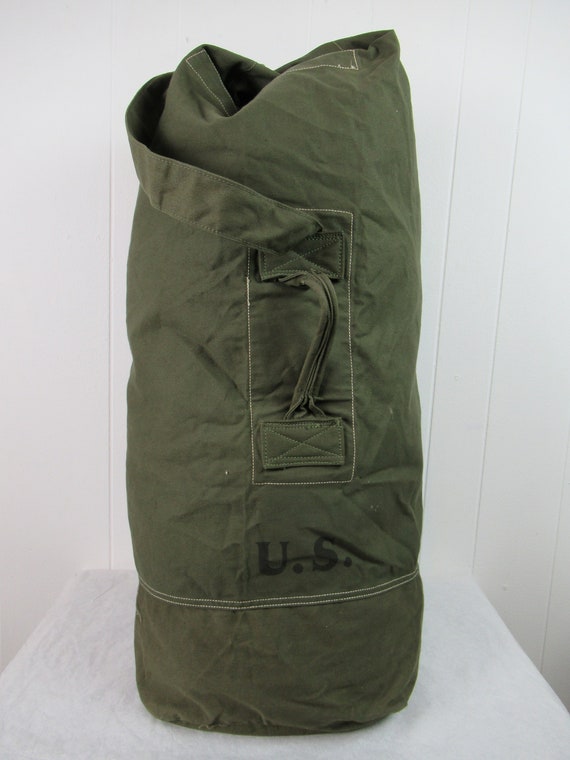The image portrays a detailed and reinforced U.S. Army duffel bag of a dark olive green color standing vertically on a white platform or table. The bag features a cylindrical shape and is made of durable, wrinkled fabric with prominent white stitching throughout, suggesting strong reinforcement, especially around the handles. There are two handles: a smaller one attached to the top middle and a larger strap extending across the top. Beneath the smaller handle, the letters "U.S." are conspicuously painted in black. The bag appears closed but has visible folds indicating the opening at the top. It is set against a backdrop of a white, grooved wall, likely paneling.